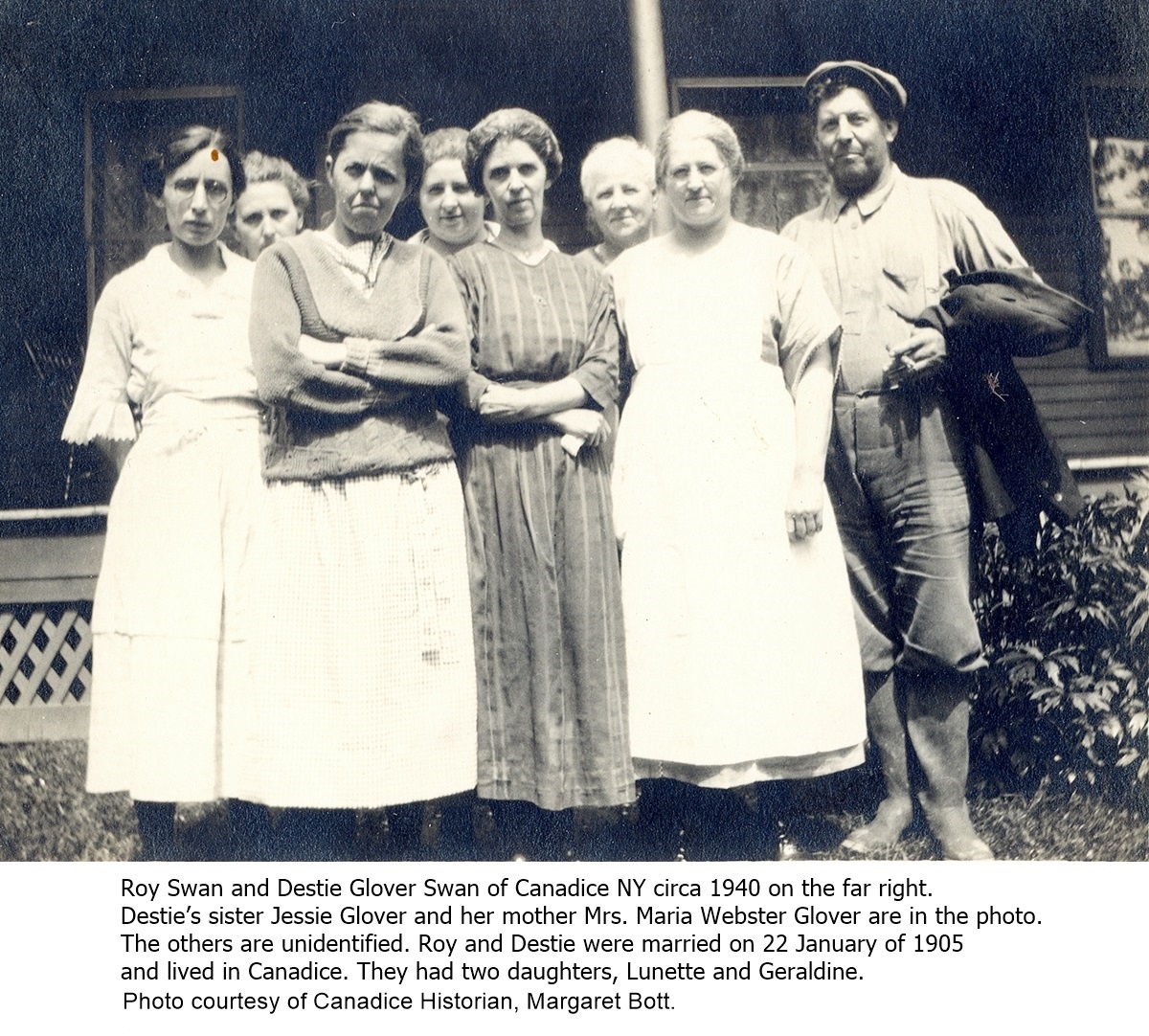This black and white photograph, taken circa 1940, shows a group of eight people standing in front of a house, identified by the text beneath as Roy Swan and Dusty Glover Swan of Candace, New York. Roy Swan is the sole man, positioned on the far right, wearing a cap and holding a jacket over his arm. Beside him in historical context is Dusty's sister, Jessie Glover, and her mother, Mrs. Maria Webster Glover. While the identities of the remaining group members remain unknown, the photograph captures seven women and one man in total, arranged with four women in the front row and three behind. Some women don white dresses while another sports a sweater, with two front-center women crossing their arms sternly. None of the individuals, including Roy, are smiling, contributing to the photograph’s austere tone. The home in the background features visible windows, a porch, some shrubbery, and an unidentified pole. The historical image is authenticated by Canada's historian Margaret Lott, detailing that Roy and Dusty were married on January 22, 1905, resided in Candace, and had two daughters, Lynette and Geraldine.